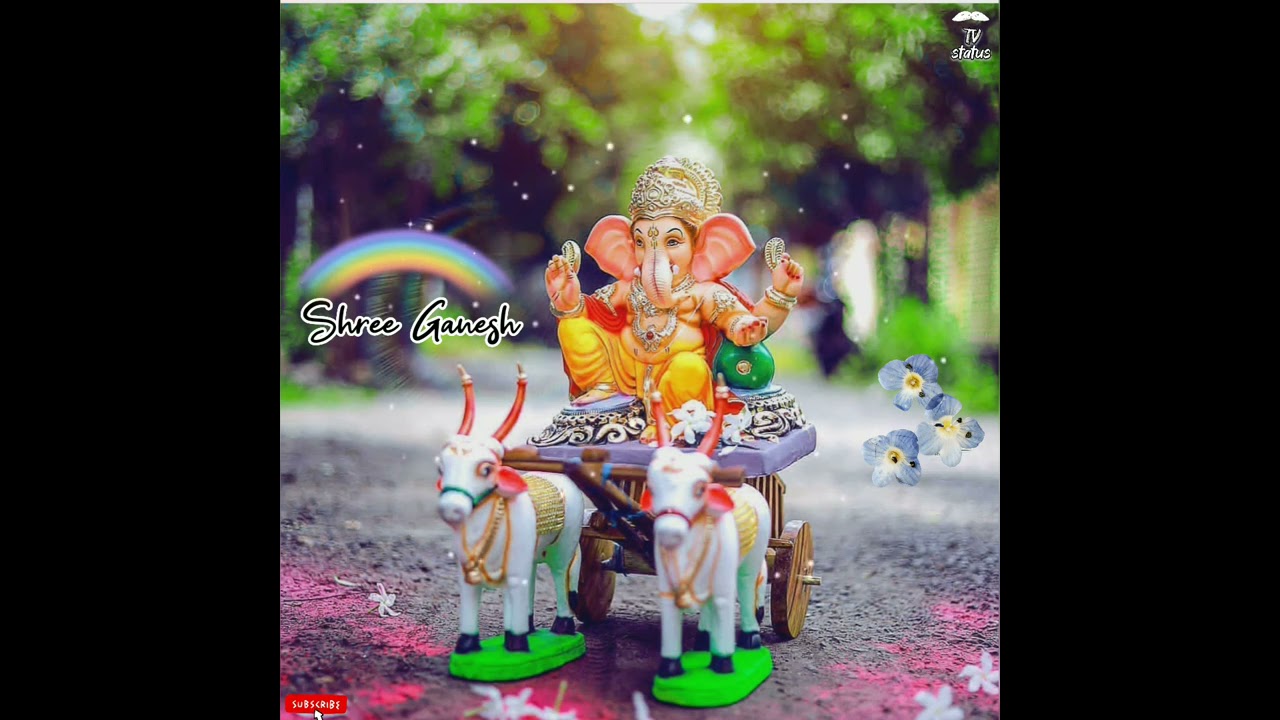This detailed image showcases a close-up shot of a figurine depicting the Indian deity Lord Ganesh, merging human and elephant features. Ganesh, adorned with a golden crown and ornate decorations on his forehead, has pink ears, human hands, and is dressed colorfully in yellow pants and a red scarf. He is seated on a purple surface atop a two-wheeled wooden cart, which is being pulled by two white goats with golden saddles and chains around their necks. The cart itself stands on light green platforms. The background features a lush, green landscape with trees and natural sunlight streaming through, along with an asphalt or dirt path. Above the figurine, there is a rainbow motif, and a handwritten-style caption on the left side of the image reads "Shree Ganesh" (S-H-R-E-E-G-A-N-E-S-H) in black and white. The scene is also adorned with pink flowers or perhaps pink chalk, adding to the vivid and whimsical aesthetic.